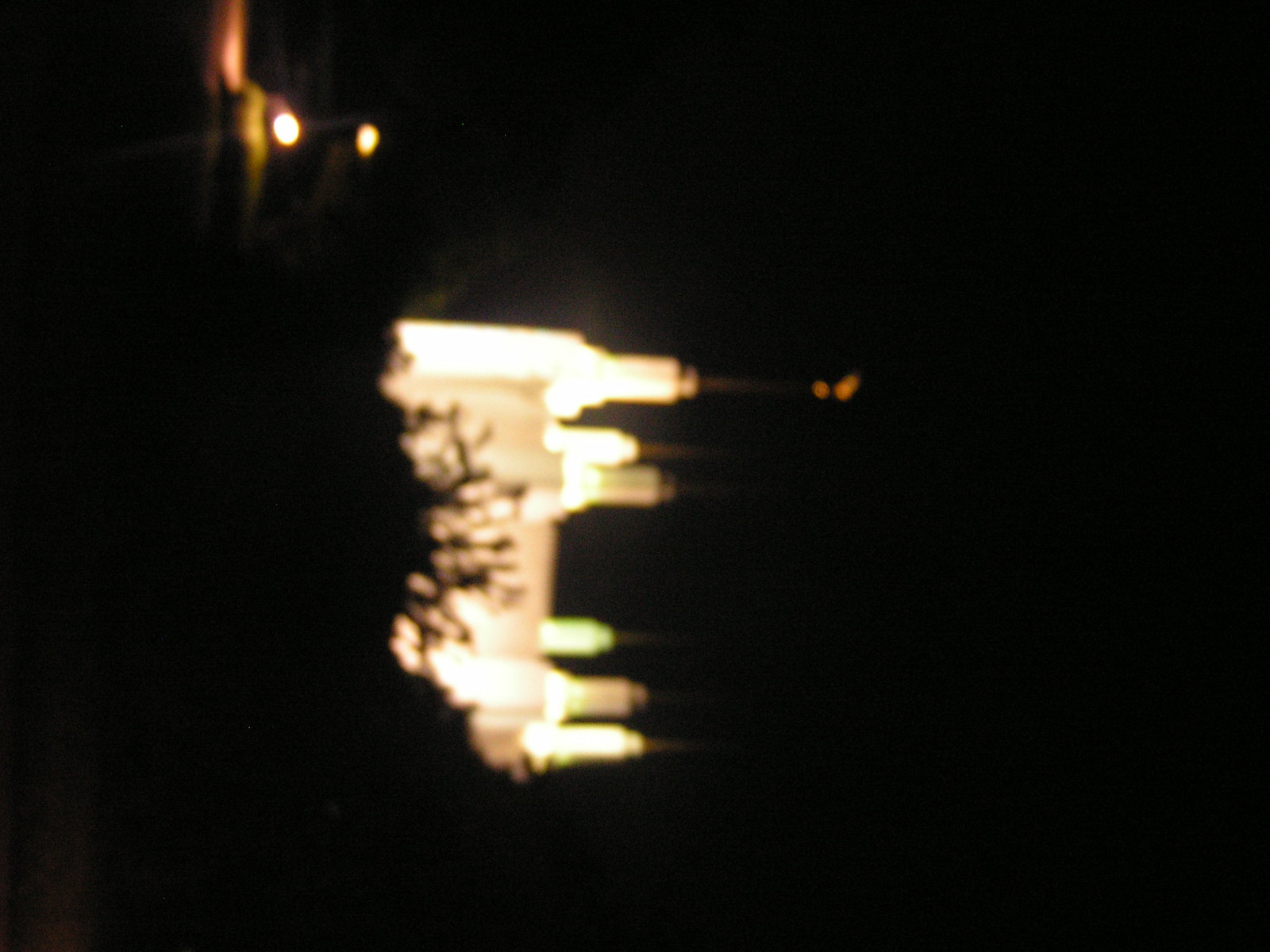The image is a blurry, 4x6 photo predominantly dark, likely taken outdoors at night with a completely black background. Centered in the mid-ground is a brightly illuminated structure, possibly a building or castle, featuring indistinct elements that might be turrets or parts of adjacent buildings, suggesting a skyline. The overall impression is that the image is sideways, as indicated by the orientation of what appears to be a sideways bush or tree and a pole with a flag. The blurriness and the bright illumination make it difficult to clearly identify the exact details or confirm the exact nature of the structures.